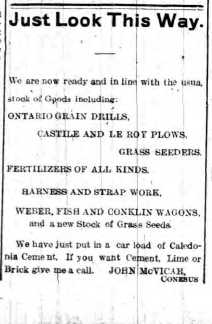The image is an old newspaper advertisement with a white background, featuring several black lines that give it a damaged appearance. It is bordered by black lines with additional paper visible beyond the border. At the top of the ad, the bold phrase "Just Look This Way" is printed in large black text. Below it, there's smaller and partially illegible text, followed by clearer advertising content. The advertisement declares, "We are now ready and in line with the usual stock of goods," listing items such as Ontario Grain Drills, Castile and Laurent Plows, Grass Seeders, Fertilizers of all kinds, Harness and Strap Work, Weber Fish and Conklin Wagons. It mentions a new stock of "We have just put in a carload of Caledonia cement." The ad also states, "If you want cement, lime, or brick give me a call," and is signed by John McVicar accompanied by another illegible word. The detailed layout and context suggest that it's an advertisement related to farm and building supplies.